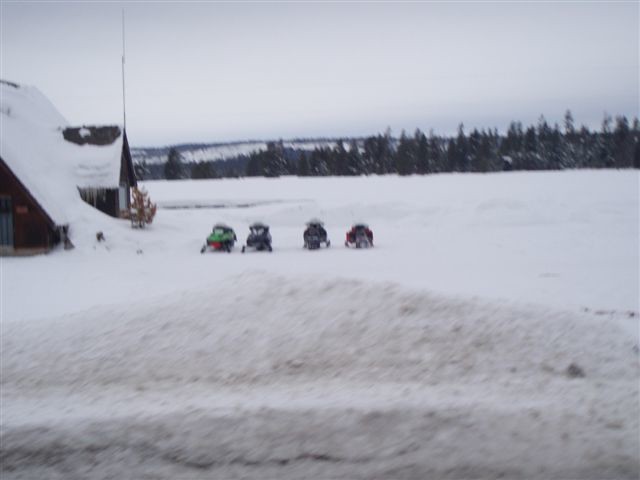A slightly blurry, landscape-oriented color photograph captures a wintry outdoor scene. The open, snow-covered land is marred by slightly off-white snow drifts at the forefront, which appear to have dirty beige patches. Dominating the middle of the image are four lined-up vehicles; although difficult to discern due to the image's graininess, they likely include snowmobiles and possibly a toboggan on the far right. An A-frame wooden cabin, its roof heavily blanketed with snow, anchors the left side of the frame. The cabin's facade showcases wood paneling amidst the encroaching snow. In the background, a dense row of dark evergreen trees stretches across the horizon, contrasting with the wintry sky above. The sky itself is predominantly a mix of white and grey clouds, though an elusive hint of blue peeks through the lower right corner. The backdrop also hints at a snow-covered mountain range, adding depth to the serene, yet somewhat indistinct wintry landscape.